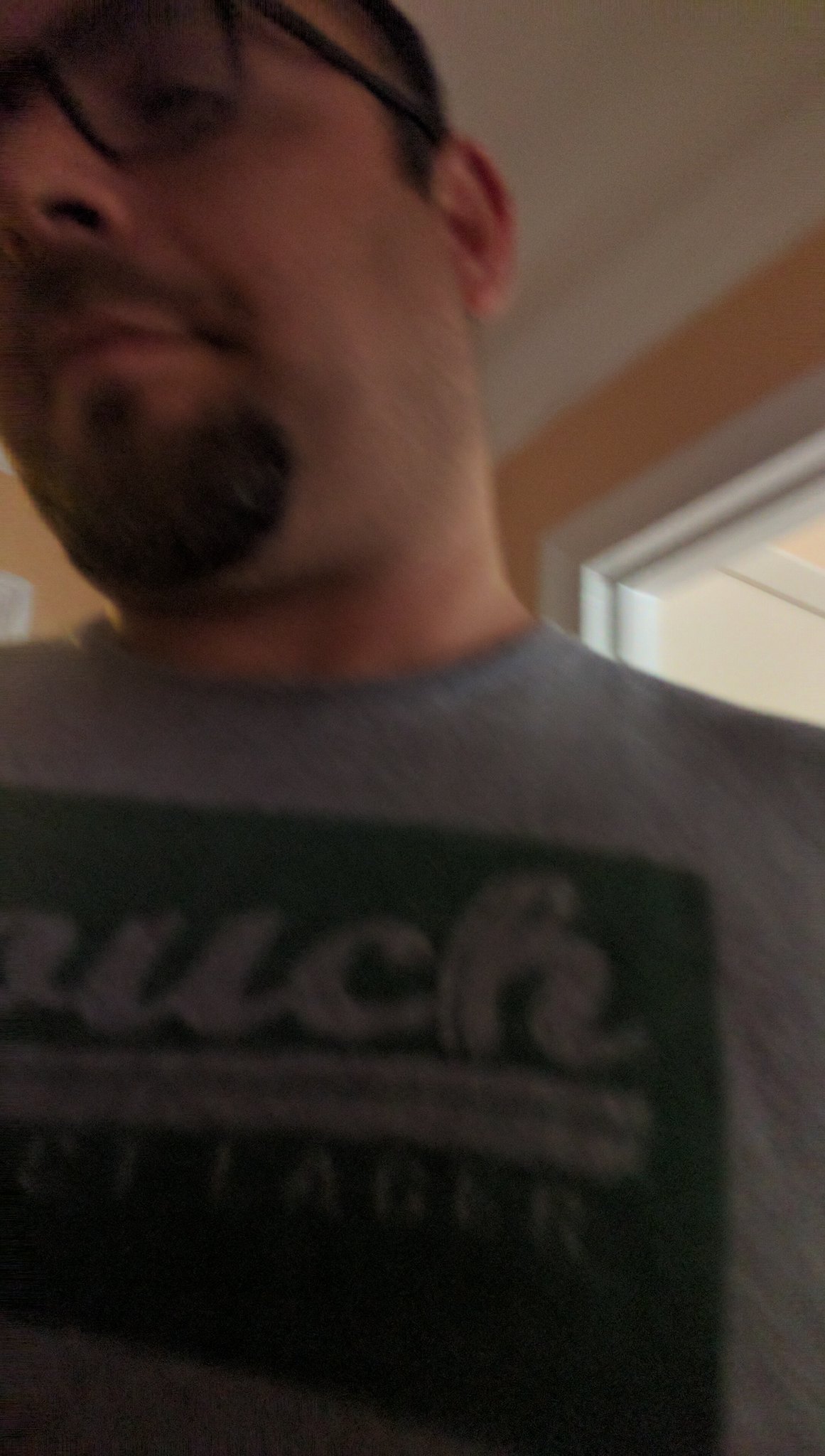This image captures a blurred close-up of a Caucasian male. He is wearing black-rimmed glasses with black temples, and has short dark brown hair, a small mustache, and a short brown beard, forming a goatee. His head appears cut off by the top-left corner of the vertical, rectangular photo, suggesting it was taken from a low angle, likely with an iPhone. The man is looking to the left and moving in that direction, which causes the blur. He is dressed in a dark gray crewneck t-shirt featuring a green logo that includes the letters "U-C-H" and the word "logger" in thinner gray script beneath a gray rectangle. Behind him, the background shows a white ceiling with white molding, meeting a peach-colored wall. There is an open doorway with a white wooden frame leading into a cream-colored room. Additionally, a partial view of another white doorframe is visible to the left.